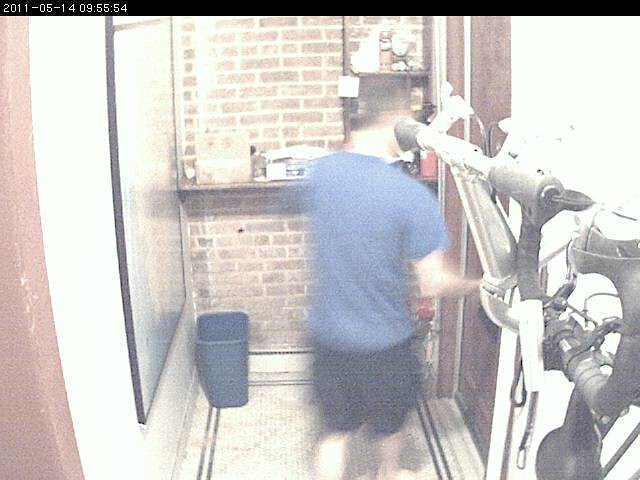This security camera still, dated May 14, 2011, at 09:55:54, captures an indoor scene with a man in the center. The man, a white male, is slightly blurred as he moves, dressed in a medium blue short-sleeved T-shirt, black knee-length shorts, and a black cap. His back is turned towards the camera. The setting features a brick wall with red bricks and white cement in the background. To the left of him, there is a white wall with a framed picture or mirror and a blue-gray trash bin underneath. In front of the man is a storage shelf that holds various items, including bottles that look like spray cans. To his right, there's an exercise machine with cables and pipes. At the bottom left of the image, a wooden door frame suggests another room off to the side. The floor appears to be white tile. The image has a black bar at the top displaying the timestamp.